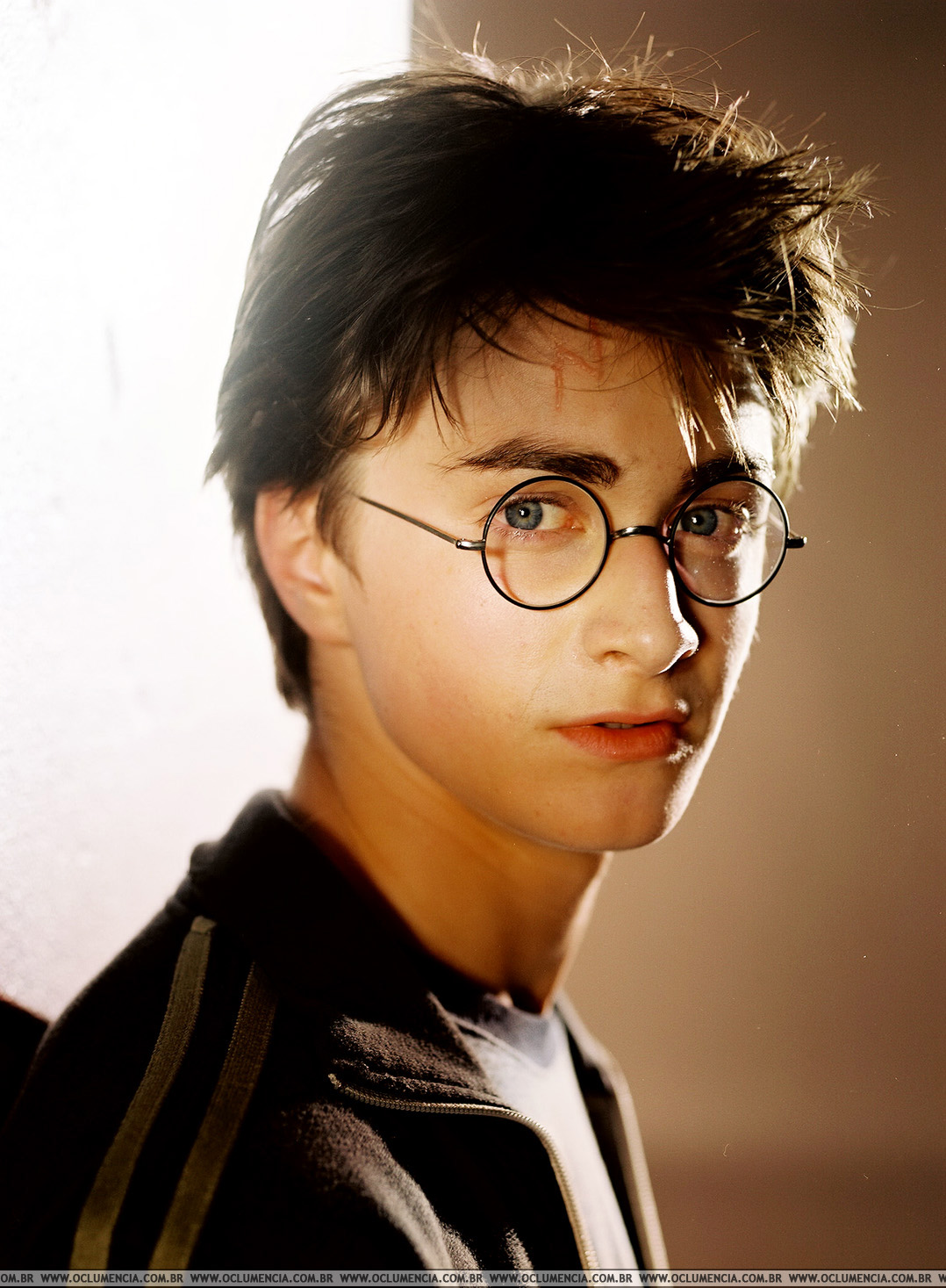This professionally-taken color photograph features a young Daniel Radcliffe, the actor best known for his role as Harry Potter. He is centrally positioned in the image, gazing intensely at the camera with his mouth slightly open and an expression of seriousness on his face. Radcliffe sports his iconic Harry Potter look, complete with round, wire-rimmed glasses and slightly messy brown hair. He is dressed in a black zippered sweatshirt with two stripes down the shoulders. The background is blurred, with a gradient from bright white on the left to tan-brown on the right, containing no discernible details or text except for an indistinct, tiny line at the very bottom. The overall color scheme includes shades of peach, orangish pink, black, white, green, brown, and gray, contributing to the professional and polished aura of the shot.